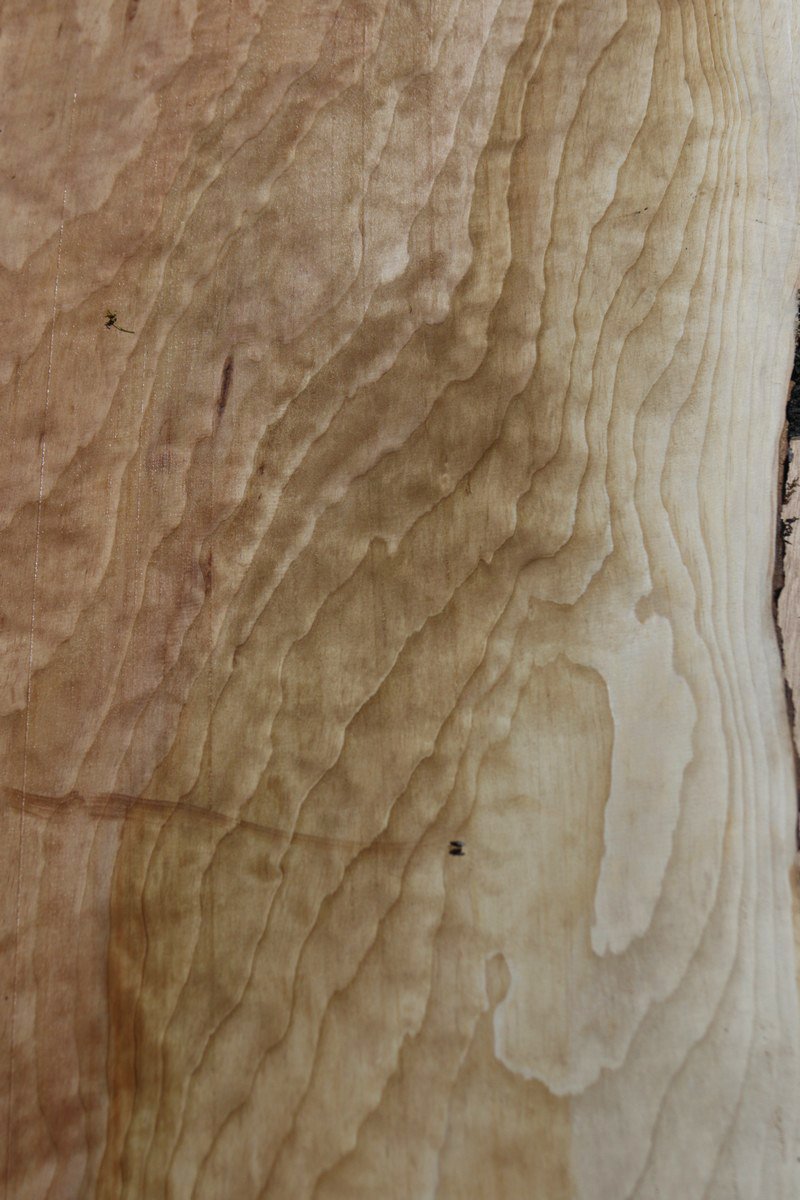This detailed image showcases a close-up of a smoothly milled and sanded piece of wood, presenting an intricate grain pattern that resembles a fingerprint. The wood surface starts with a dark beige color on the left, progressively transitioning to a lighter beige and almost white on the right. The grain pattern features a series of light brown, squiggly lines that traverse from top to bottom, creating a visually dynamic, watermark-like effect. Small black specks are sporadically scattered across the wood, adding subtle texture. In the far right section, a thin strip of what resembles bark can be seen, contrasting with the smooth, patterned wood that dominates the rest of the image. The wood appears flat, indicating careful milling and sanding, with no visible bumps. Overall, the image captures the natural beauty and detailed grain patterns of the wood, which may be part of a larger furniture piece, like a table.